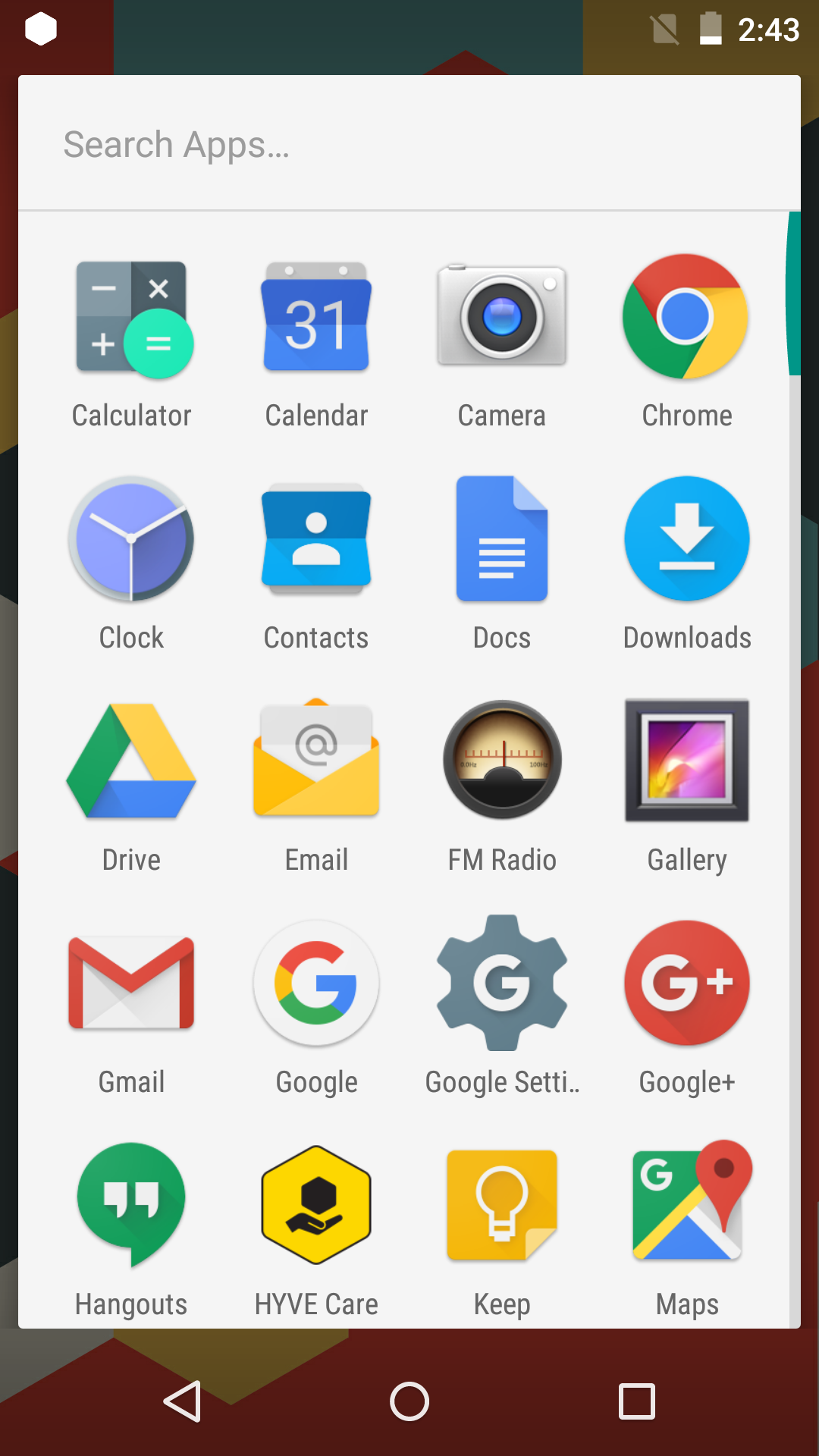This screenshot captures the app drawer of an Android phone. At the top right corner, the time is displayed as 2:43, and the battery level is approximately 10%. Directly below this, there is a search box labeled "Search apps."

The app drawer is set against a clean, white background, and each app is represented by its respective icon and label. The apps are organized starting from the top left corner, moving to the right and then downwards. The visible apps include:

1. Calculator
2. Calendar
3. Camera
4. Chrome
5. Clock
6. Contacts
7. Docs
8. Downloads
9. Drive
10. Email
11. FM Radio
12. Gallery
13. Gmail
14. Google
15. Google Settings
16. Google Plus
17. Hangouts
18. Hyve Care
19. Keep
20. Maps

Most of these are default Google applications. Notable exceptions include "Email," likely the stock email app provided by the device manufacturer (such as Samsung or Motorola), "Hyve Care," which seems to be a specific app possibly related to device maintenance or support, and "FM Radio," which may be pre-installed by the manufacturer.